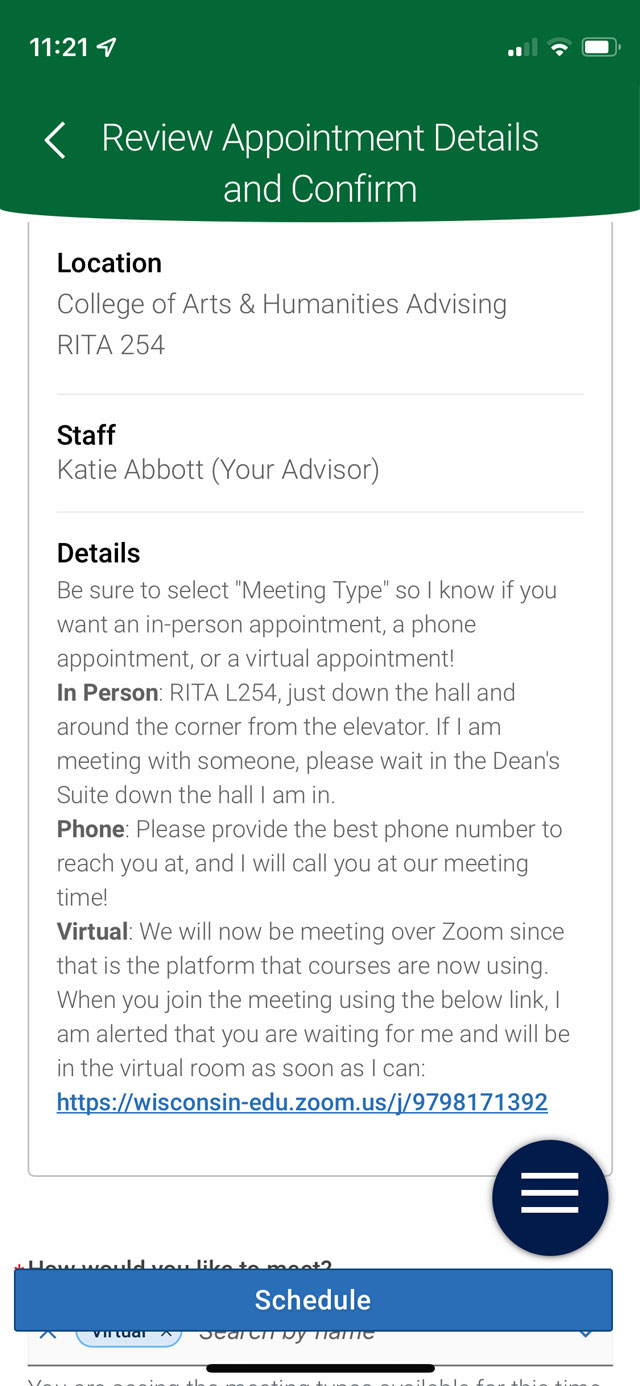Screenshot of a phone displaying an appointment confirmation screen. The green banner at the top shows the time, "11:21," and signal strength with two out of four bars filled. To the far right, there is an almost full battery icon. The main heading reads "Review Appointment Details and Confirm" on a white background. The subsequent sections provide detailed information:

- **Location:** College of Arts and Humanities, Advising, RITA 254.
- **Staff:** Katie Abbott, Your Advisor.
- **Details:** 
   - **In-Person:** Indicates the in-person meeting location at RITA L254, noting it's down the hall and around the corner from the elevator, with a request to wait in the dean's suite if the advisor is meeting with someone else.
   - **Phone:** Requests the best contact number for the advisor to reach the student at the scheduled meeting time.
   - **Virtual:** States that meetings will be conducted over Zoom, providing a detailed explanation about the use of Zoom for virtual meetings, mentioning that the advisor is alerted once the student joins with the provided link.

At the bottom of the screen, there is a blue "Schedule" button.